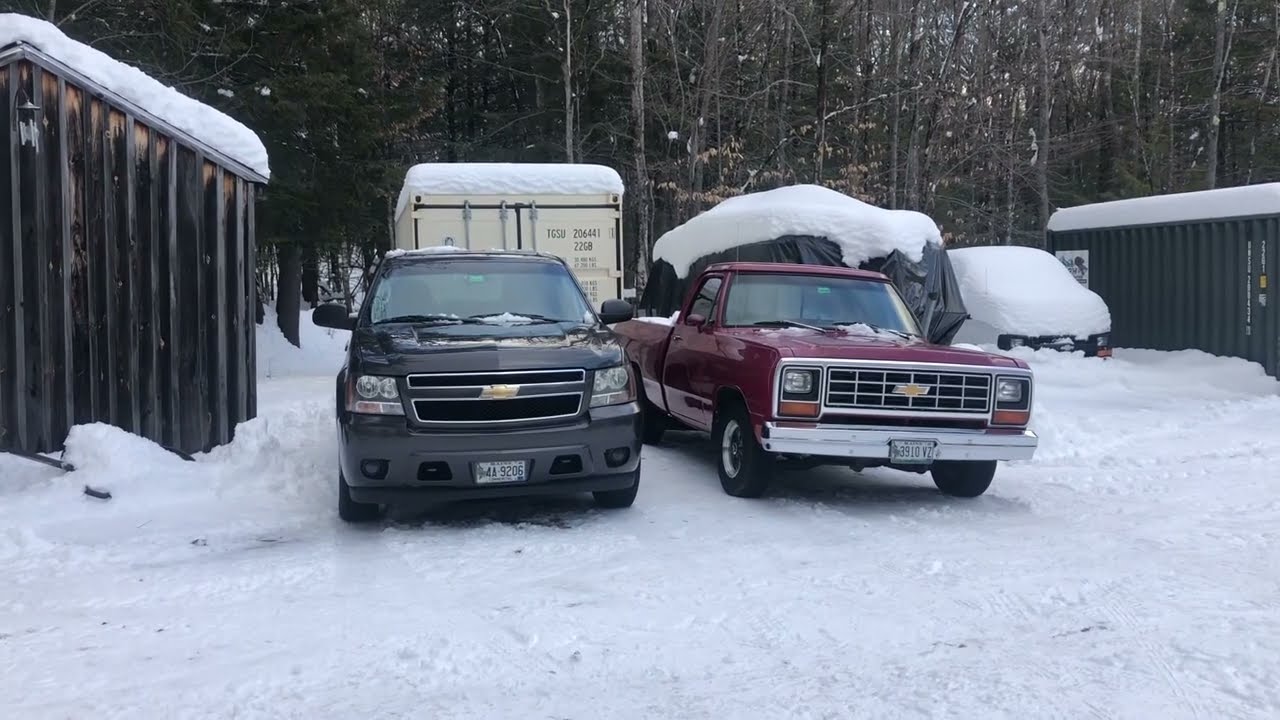Amidst a snowy landscape, the scene showcases two Chevrolet pickup trucks parked side by side. The truck on the left is a dark gray, newer model, bearing a Chevrolet emblem on its grille and a mostly white license plate. It's lightly dusted with snow. The truck on the right is an older, maroon model with a silver bumper and a similar Chevy emblem, also topped with a light layer of snow. Behind the trucks looms a light cream-colored storage container, its roof burdened with a solid layer of snow. To the right of the container, a black plastic covering lies on the ground, also capped with snow. A van, barely visible under its snowy blanket, and another green-colored container occupy the far right. On the far left, a small wooden building, resembling an outhouse, stands with snow frosting its roof. The backdrop consists of a dense row of trees, where the mix of green evergreens and bare, brown deciduous trees creates a variegated tapestry. This picturesque scene, blanketed in snow thickly covering the ground and every surface, captures a quintessentially wintery moment.